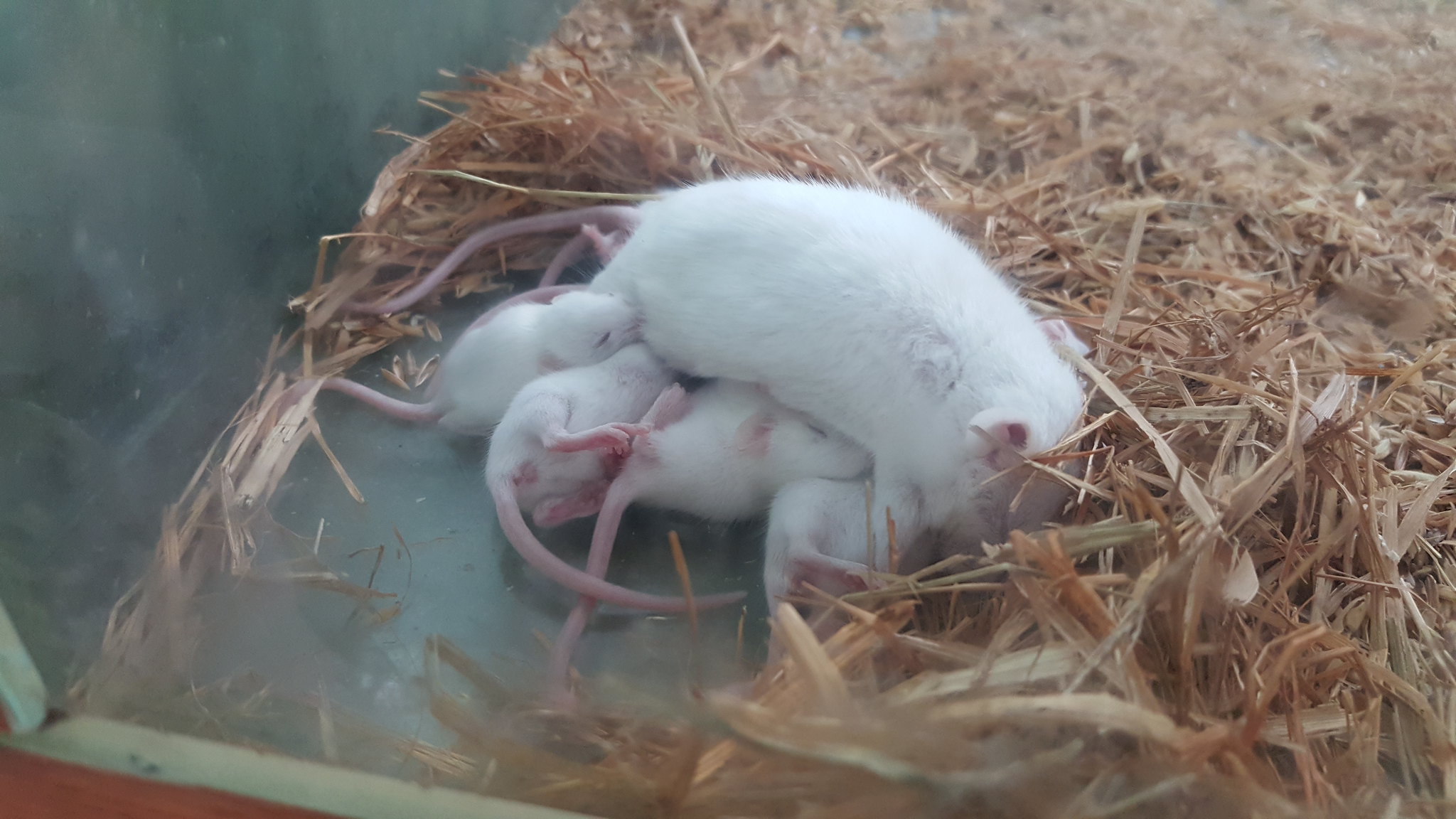The image shows a mother mouse, white with a pink tail, laying on her side in a glass enclosure. Four baby mice, also white with pink tails, are either nursing or resting beneath her belly. The baby mice are nestled closely to the mother, and their heads are mostly obscured by her body. The enclosure's floor is a flat, gray surface scattered with yellow hay. One of the enclosure's side walls features a pink or red-colored paint. The scene gives an impression of a nurturing family moment within the secure confines of the enclosure.